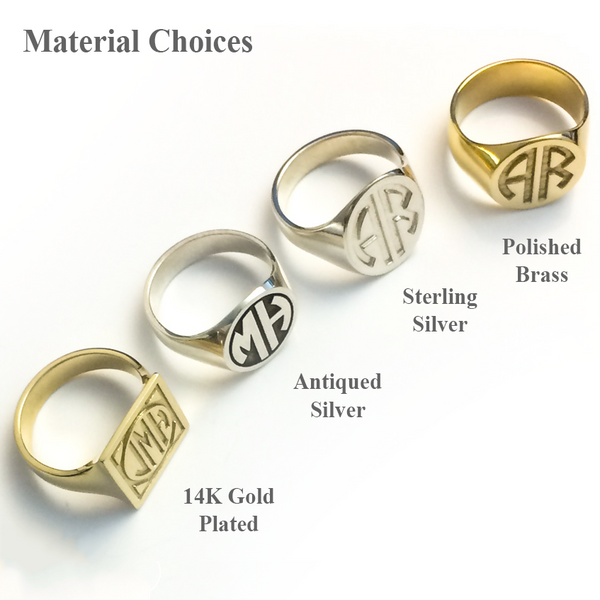The image showcases a collection of four distinct signet rings arranged in a row against a pristine white background, likely designed for an advertisement. In the upper left corner, bold black lettering spells out "Material Choices." Each ring is meticulously labeled with its respective material and engraving. From the bottom up: the first ring is labeled "14K Gold Plated" and features the initials "JMH"; the second ring is an "Antique Silver" circular signet with the initials "MH"; the third ring, also round, is marked "Sterling Silver" and displays the initials "AR"; and the topmost ring, similarly round, is noted as "Polished Brass" and also bears the initials "AR." This detailed display provides potential buyers with a clear visualization of the available material and engraving options for the signet rings.